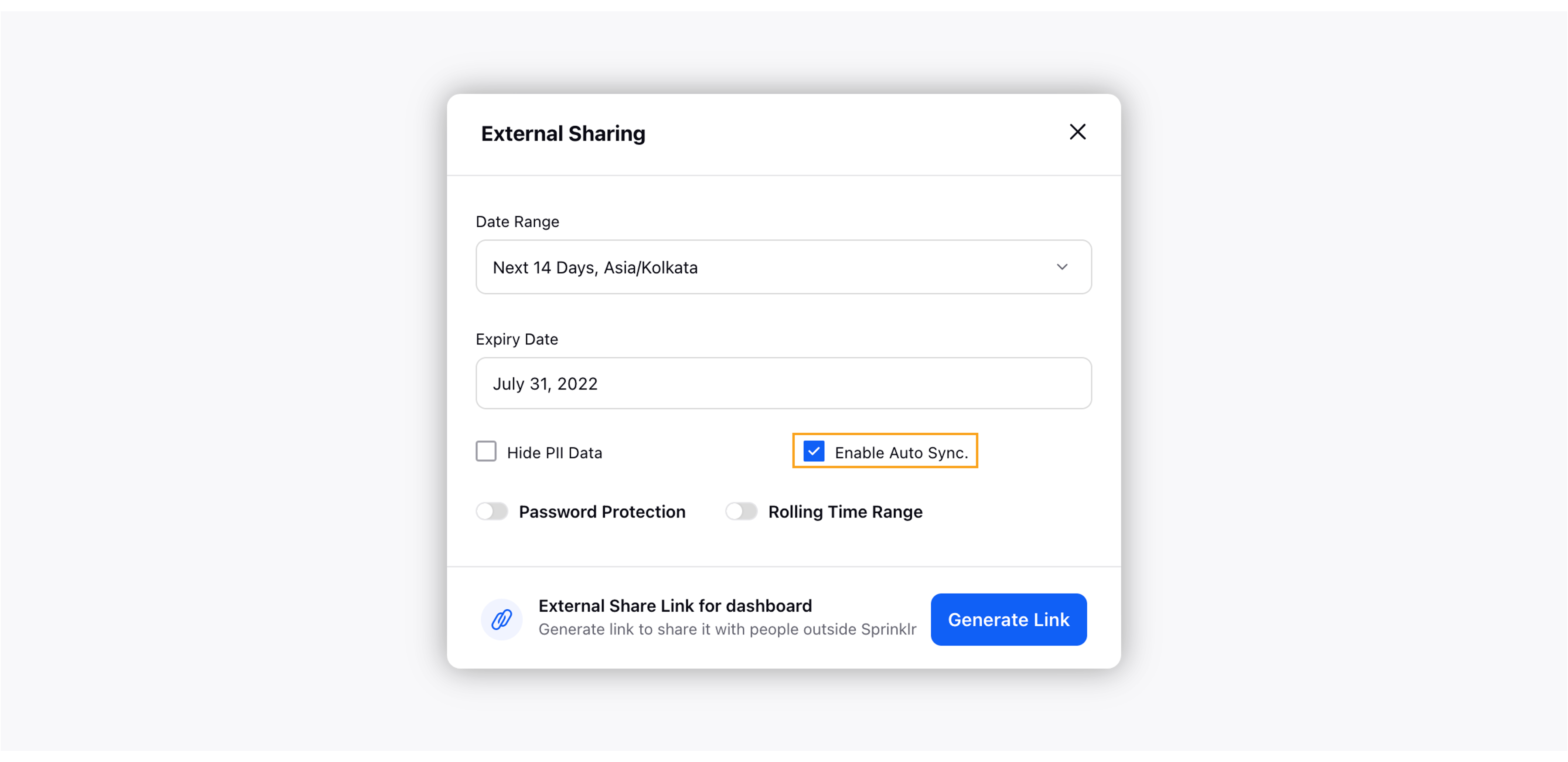In the image, there is a white dialog box titled "External Sharing." Below the title, users can select a date range. The current option chosen is "Next 14 days," with the regional settings specified as "Asia/Kolkata". The dialog also displays an entered expiry date, which is July 31st, 2022. Beneath the date options, there is a selected checkbox labeled "Enable Auto Sync." Another option, labeled "Hide PH Data," remains unselected. At the bottom of the dialog box, there is a prominent blue button labeled "Create to Generate a Link."